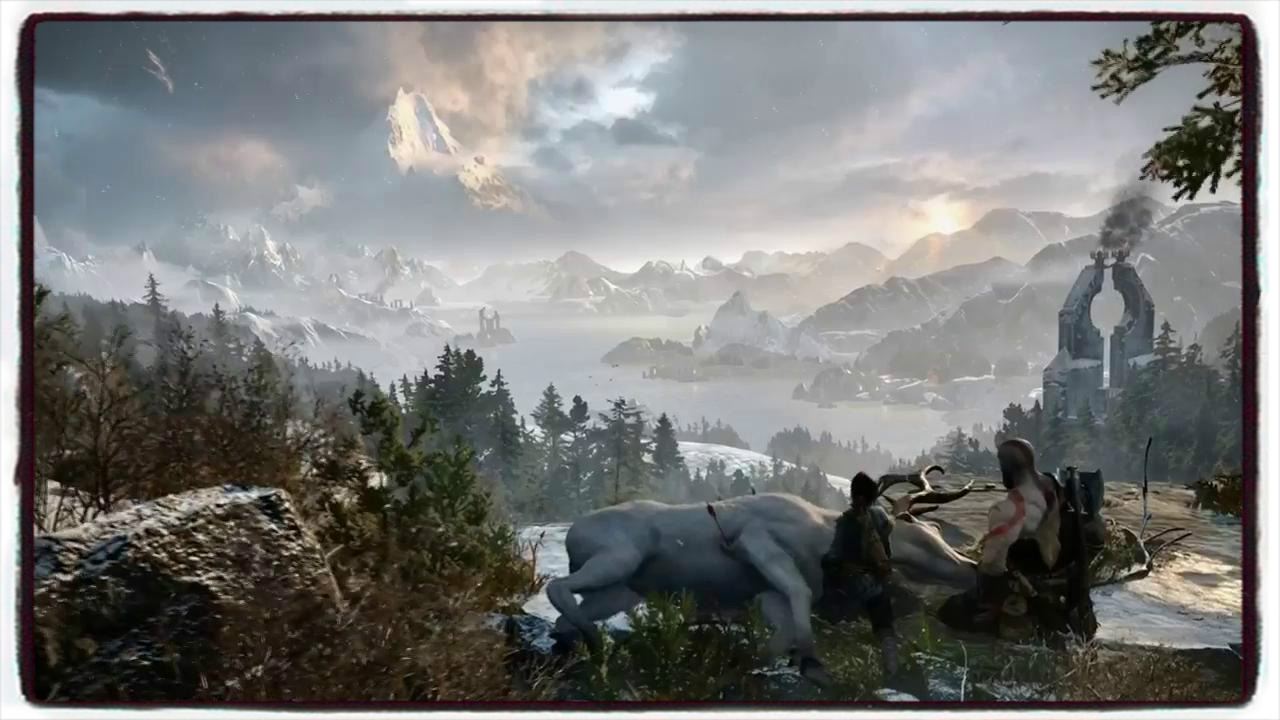The image appears to be a meticulously crafted 3D digital rendering, possibly derived from a video game or digital art, with a distinct fantasy theme. Enclosed within a rich brown border, the scene evokes a sense of myth and legend, reminiscent of the atmospheres found in "God of War."

On the right-hand side of the image, a muscular man is depicted kneeling somberly. His notable physique is adorned with red tattoos that trail down from the back of his head to his chest, suggesting a character steeped in warrior tradition. Beside him stands another figure dressed in an archer's outfit, lending an air of readiness and tension to their presence.

Prominently lying on its side in the foreground, a majestic white stag with golden antlers lies still, a poignant arrow protruding from its body, indicating its recent death. This fallen creature adds a narrative depth, hinting at a significant event that has just transpired.

The backdrop seizes attention with its breathtaking ascent of mountainous terrain, merging into what appears to be a divine realm, possibly symbolizing Mount Olympus. To the right stands an enigmatic stone structure with a large circular aperture, adding a mystical architectural feature to the landscape. Below the mountains, a serene lake occupies the valley, contributing a tranquil yet solemn touch to the overall composition.

The meticulous details and dynamic positioning within the scene suggest a moment of profound significance within a fantastical world, blending elements of mythology, tension, and solemn beauty.